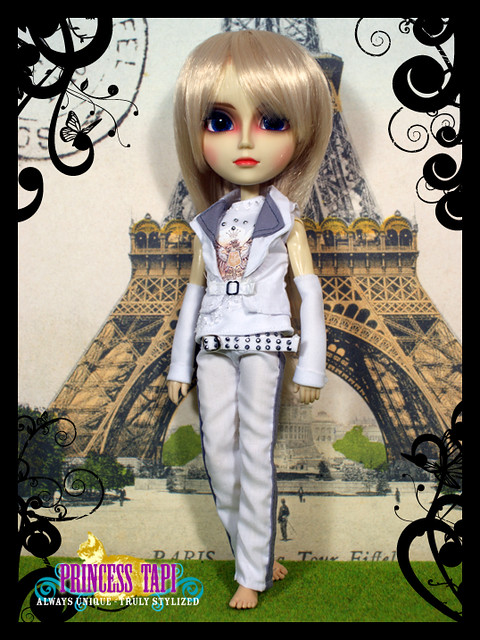The image features a detailed doll dressed in a stylish white outfit. The ensemble includes a white vest, white sleeves on both arms, white pants with a black stripe down the side, and a white belt adorned with black dots. The doll, barefoot and standing on a grassy surface, has striking blonde hair and appears heavily made up with noticeable makeup and vividly painted lips. She is positioned before a backdrop illustrating the Eiffel Tower, which transitions from a tan base to a silver upper structure. The photograph is bordered by a black swirl design, and in the lower left corner, the text "Princess Tappy" is inscribed in purple, accompanied by the phrase "Always unique, truly styled."